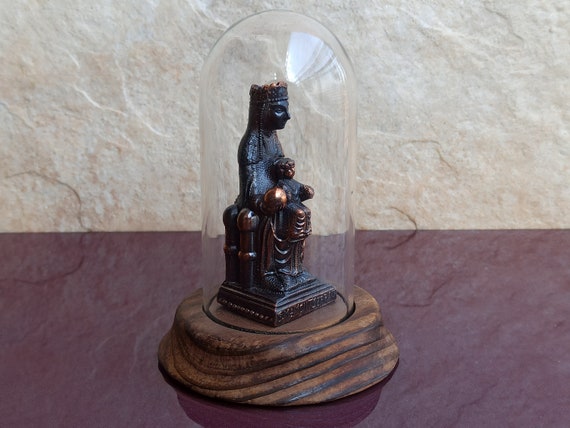The photograph features a detailed bronze figurine of what appears to be Mary holding a child, encased in a clear glass dome. The figurine, presented in a three-quarter view angle to the right, showcases Mary seated on a low-backed, intricately sculpted throne, adorned with a peaked crown and a flowing robe. Her long hair cascades below her shoulders, and she tenderly holds an infant child on her lap, whose legs are visible. The entire set-up rests on a round walnut base, placed on a dark, purplish-burgundy marble top. Behind this scene is a white stone or stucco wall, adding contrast to the figure's dark tones and the marble surface. The image is brightly lit, providing clear visibility of all the intricate details and textures of the sculpture and its surroundings.